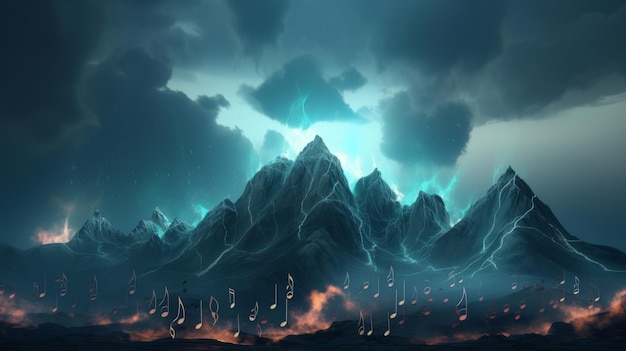The image is a striking piece of computer-generated art featuring a cluster of dark, steep mountains with jagged, pointy peaks. These peaks seem to move in unison and are accented by bright, glowing blue streams resembling rivers or electricity cascading down their slopes. Towards the base, an orange, misty aura with fiery tones suggests lava flows, and bizarrely, musical notes dance across this fiery expanse from left to right. The sky above is turbulent with large, dark clouds, and dramatic lightning discharges. Over the center of the mountains, a brilliant blue light emanates, creating a vortex of illumination that fades as it radiates outward, contrasting against the gradated backdrop that shifts from dark at the horizon to lighter near the mountain tips.